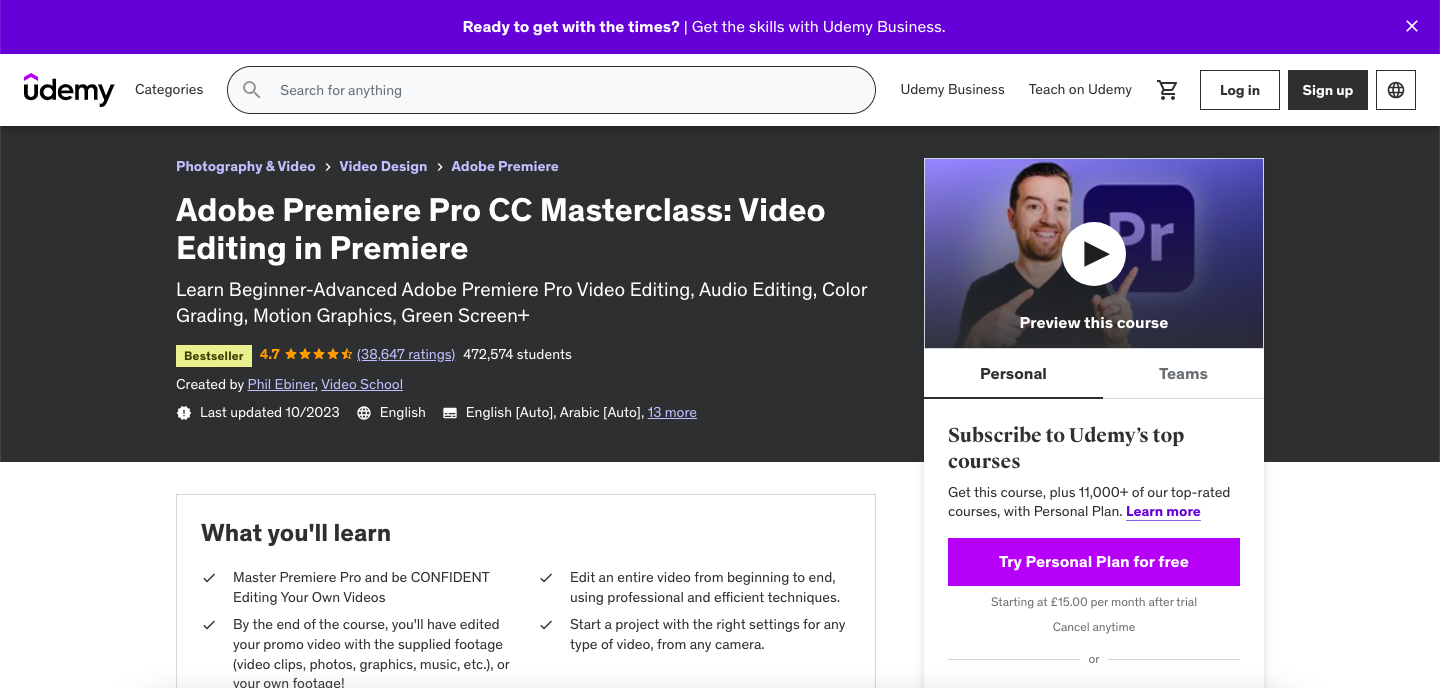The image is a screenshot from the website Udemy, captured from a desktop or laptop display, evidenced by its elongated proportions. In the upper left-hand corner, the Udemy logo is prominently displayed in lowercase letters. Adjacent to the logo, there's a search box followed by several clickable text links including "Login," "Sign Up," and a shopping cart icon.

Below this navigation bar, the screenshot highlights a specific course available for purchase. The course is presented against a dark grey background, with the title in white text: "Adobe Premiere Pro CC Master Class: Video Editing in Premiere." The subtitle elaborates, "Learn beginner to advanced Adobe Premiere Pro video editing, audio editing, color grading, motion graphics, green screen techniques, plus more."

This program is tagged as a "Best-seller" and boasts a rating of 4.7 stars out of 38,547 ratings. It was last updated in October 2023. To the right of the course details, there is a clickable video preview thumbnail, inviting users to watch a brief introduction to the course.